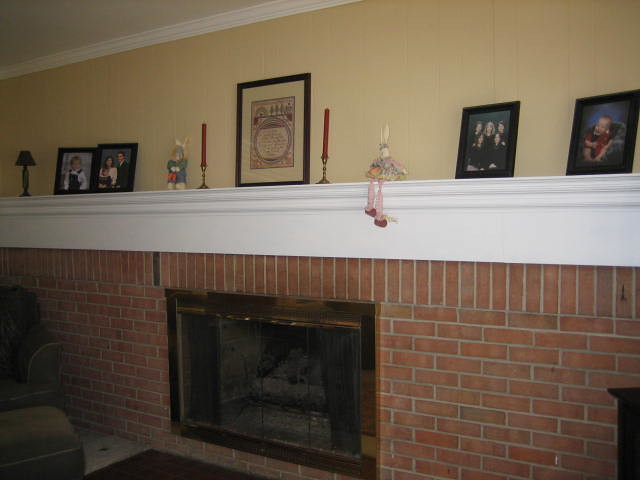An indoor color photograph captures a fireplace in a home. The fireplace is framed by red brick, which extends halfway up the wall, transitioning to a wooden shelf painted white that protrudes about six inches. The shelf, or mantle, holds a collection of family photographs in black frames, with two on each side. In the center of the mantle, directly above the fireplace, is a framed sampler with a black frame and beige mat, although the details are not legible. Flanking this central piece are copper-colored candlesticks with red candles. Two stuffed bunny figures are positioned on the mantle: one with its legs dangling over the edge on the right, dressed in a tiny calico dress, and another standing upright on the left. The fireplace features a gold-colored border around its opening, which is blackened and ashy from a burnt log. The image, taken in low light, shows a slightly dark but focused scene, capturing the cozy ambiance of the room.